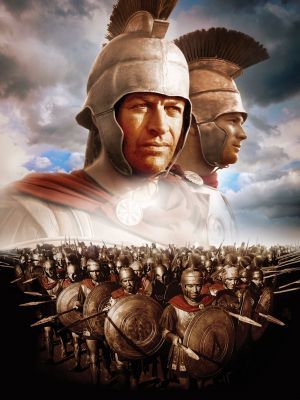The image is a heavily edited movie poster with a vertical dimension, designed to promote a film. The dramatic sky, filled with a mix of gray and white clouds, serves as the backdrop. Positioned near the top are two Roman soldiers, one facing at a 45-degree angle and the other in profile. They wear silver hammered metal helmets adorned with plumes and red capes. Below them, a vast formation of Roman soldiers stands in a battle-ready stance, each equipped with circular bronze shields and spears. The lower sections of the image are enveloped in black, enhancing the focus on the soldiers. This composition, resembling a Blu-ray cover art or a collage, captures an intense and epic atmosphere suitable for a historical film.